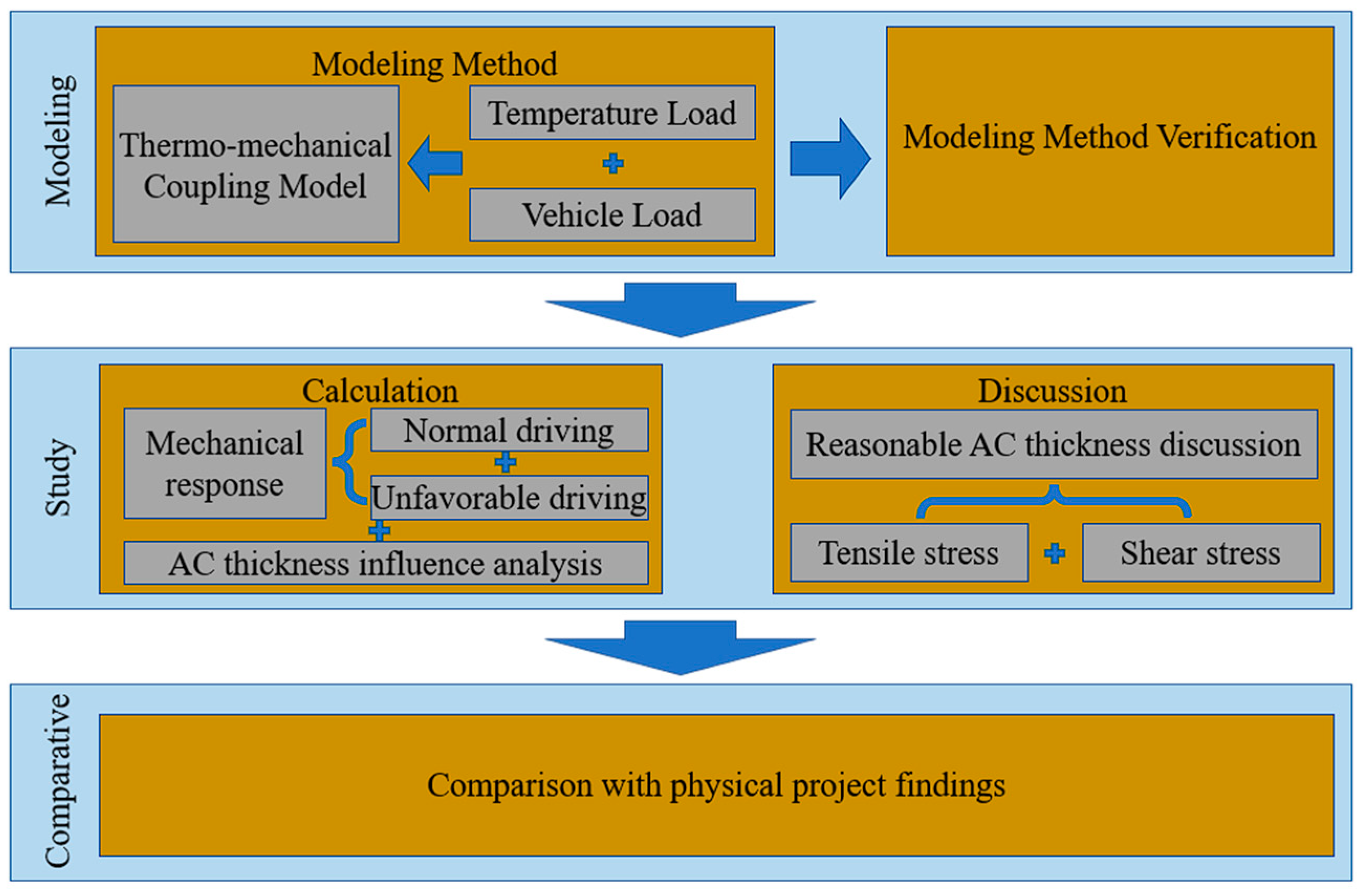The image is a detailed graphic from an old textbook, depicting a structured model in three long, evenly spaced blue rectangles with white spaces between them. The top blue rectangle is labeled "Modeling" and contains two yellow rectangles. The first yellow rectangle details the "Modeling Method," highlighting subcategories like "Thermomechanical Coupling Model" and "Temperature Load plus Vehicle Load," with a blue arrow directing towards the second yellow rectangle, "Modeling Method Verification." 

A prominent blue arrow in the white space below directs attention to the next blue rectangle labeled "Study." Within this "Study" rectangle, two yellow text boxes are present. The "Calculation" box elaborates on "Mechanical Response" with further subdivisions such as "Normal Driving plus Unfavorable Driving" and "AC Thickness Influence Analysis." Next to it, the "Discussion" box includes topics like "Reasonable AC Thickness Discussion," with brackets pointing to "Tensile Stress" and "Shear Stress."

Finally, another blue arrow leads to the bottom blue rectangle labeled "Comparative," containing an almost equally long yellow rectangle that reads "Comparison with Physical Project Findings." Each component is meticulously arranged with descriptive text in black, illustrating a comprehensive flow from modeling methods and their verification, through detailed study calculations and discussions, to comparative analysis with physical findings.